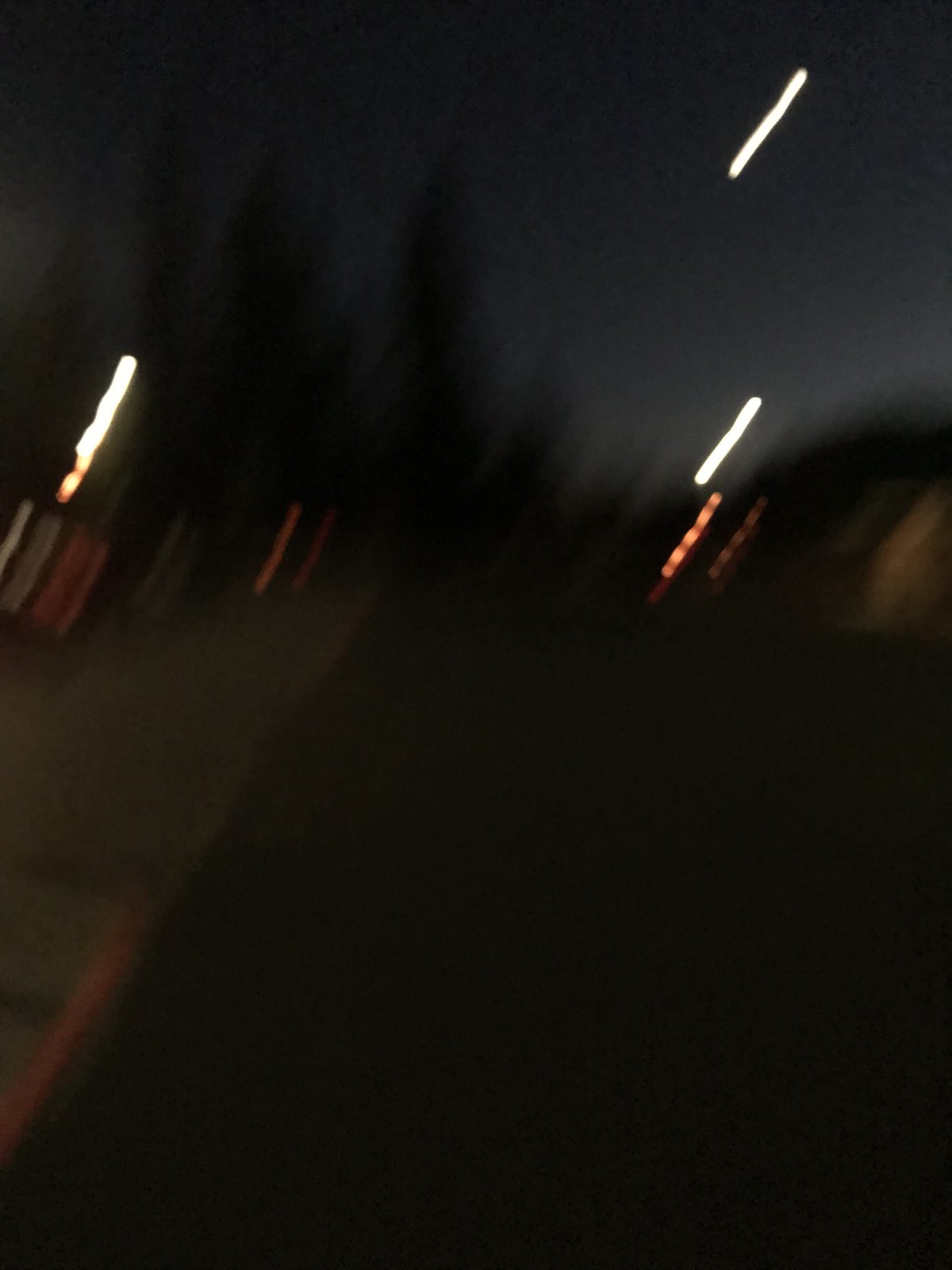The image is a very dark and blurry photograph, likely taken from a GoPro camera mounted on someone's head as they move quickly down a street. The scene is almost indiscernible due to the low light and motion blur, but you can make out some key elements. On the left side of the image, there appears to be a sidewalk, lighter in color than the pitch-black street on the right. Streaks of light punctuate the darkness, with three bright white and several red and orange lights trailing as if caught by a fast-moving camera. These lights suggest movement and add a dynamic, chaotic quality to the image. In the background, shadowy outlines of trees are faintly visible, and the sky is a very dark gray. The lower portions of the image seem to show some dimly illuminated structures and shapes, including hints of cars, although specific details are obscured by the blur. The overall impression is one of rapid motion through a dimly lit, tree-lined street at night.